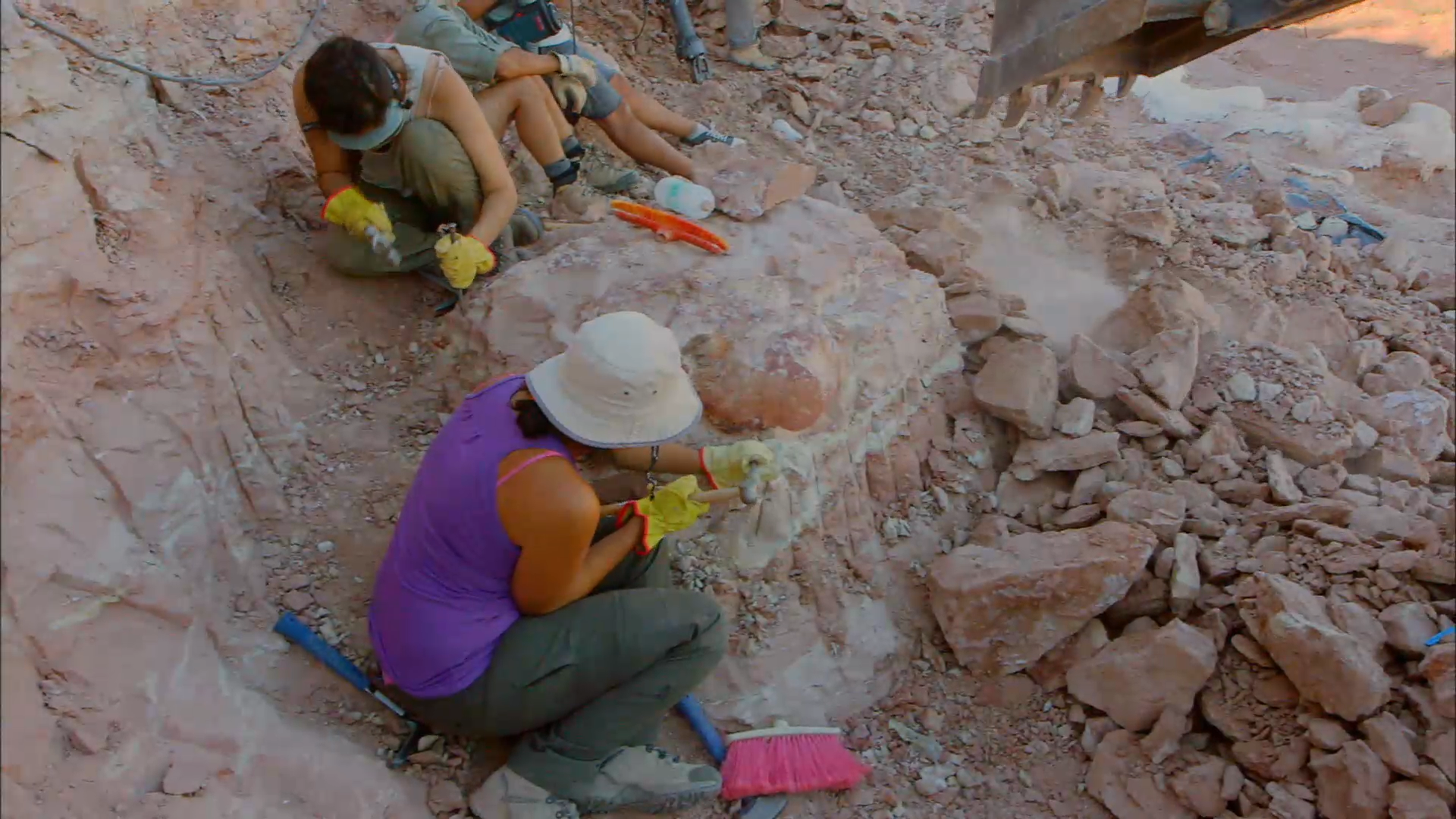In this photograph, taken at an archaeological dig site set in a rocky outdoor area, a team of people is hard at work excavating with various tools. Central in the image is a woman with dark tan skin, wearing a purple tank top that reveals a pink bra strap, grayish pants, yellow gloves with pink trim, and sneakers. She is focused, using a chisel and hammer to diligently chip away at the rocky surface. Her face and hair are shielded by a white hat. At her feet, a blue-handled hammer, the end of a brush, and a broom with pink bristles can be seen amidst the crumbled rubble. Surrounding her, a partially visible team of at least three other individuals, similarly dressed in tank tops and gloves, are also engrossed in their digging efforts. A pile of crumbled rocks and a bulldozer claw in the foreground hint at the scale of their excavation, suggesting the use of heavy machinery in addition to their manual tools to unearth whatever lies beneath.